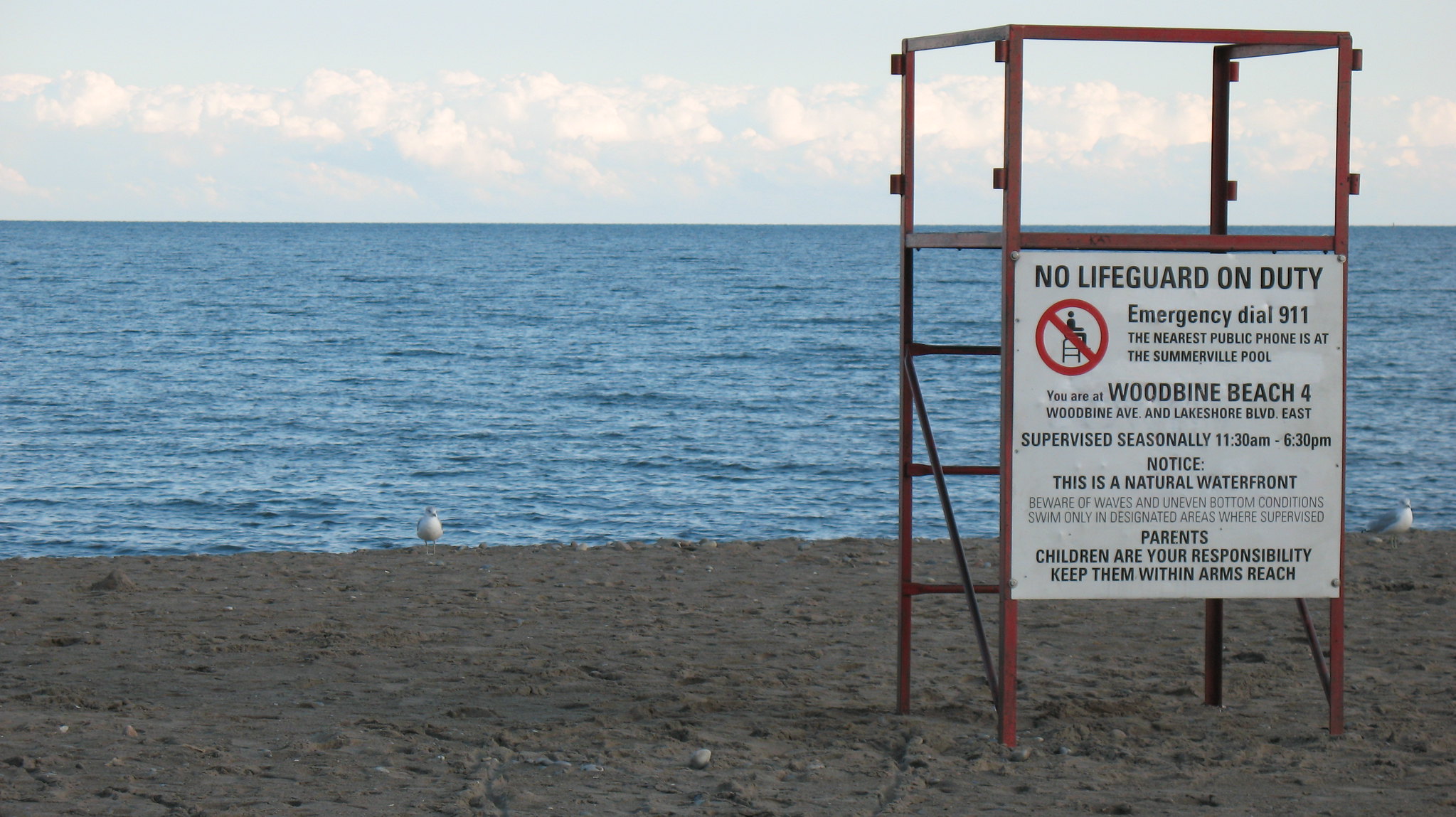The image captures a tranquil scene at Woodbine Beach 4, located at Woodbine Avenue and Lakeshore Boulevard East. In the foreground, golden sand stretches out to meet the gentle waves of the ocean. The sky above is a light blue, dotted with soft, scattered clouds. Two seagulls stand on the shoreline, one near the center of the frame and the other off to the right. Dominating the right side of the image is a lifeguard tower, constructed from thin metal poles and elevated about five feet from the sand. The tower features a sign with black text on a white background that reads "No lifeguard on duty." Below this message, the sign displays an emergency dial 9-1-1 notice and indicates the nearest public phone is located at the Somerville Pool. Additionally, the sign states, "You are at Woodbine Beach 4, supervised seasonally from 11:30 AM to 6:30 PM. Notice this is a natural waterfront; parents, children are your responsibility. Keep them within arm's reach." The sign also includes a graphic of a person sitting in a lifeguard chair, with a red circle and line through it, emphasizing the absence of lifeguard supervision.